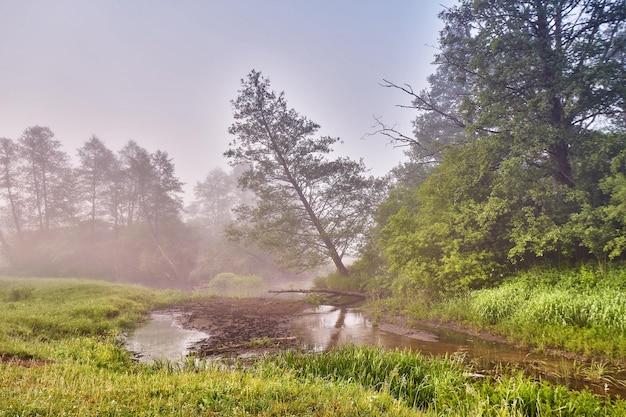The photograph captures a vibrant forested area during daytime, dominated by lush greenery and natural elements. In the foreground, a grassy embankment extends across the bottom left corner and rises slightly on the left side, tapering around a meandering river that flows through the scene. The river is moderate in width, with visible shallow areas revealing the underlying dirt. The water appears muddy, contributing to the landscape's earthy hues.

On the right side, the riverbank features light green grass and a ground layer tinged with mud. Towering pine trees densely populate both sides of the river, their green leaves painting the scenery with rich vegetation. A significant visual feature is a tall pine tree in the center of the image, precariously leaning at a 45-degree angle towards the river, looking as though it might topple over at any moment.

The backdrop reveals a slightly hazy blue sky, seemingly affected by either fog or a light mist, lending a soft grayish tint to the horizon. The overall clarity of the photograph is excellent, with the scene vividly lit by natural daylight, showcasing the landscape's lush and serene ambiance.